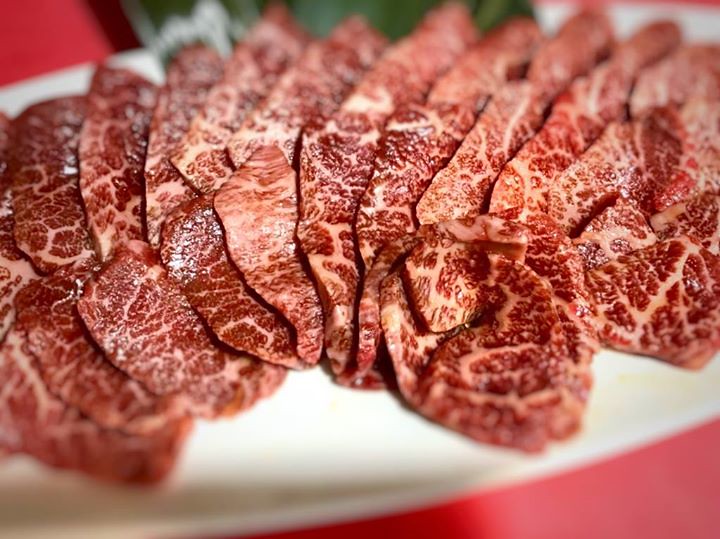The image is a close-up photograph featuring twelve pieces of lean, uncooked beef, arranged neatly in vertical slices on a slightly blurry, circular white plate. Each slice of meat varies in shades from dark red to light red, with hints of white marbling indicating the presence of fat, but overall, the meat appears to be relatively lean with minimal fat content. The white plate, extending out of the frame on both sides, is blurred, but it provides a stark contrast to the vibrant red meat. The background of the image, which also transitions to a blur towards the edges, includes hints of red, possibly from a wall or tablecloth, and green in the center, adding depth to the composition. The depiction of the beef's marbling and the clear red color suggest that it is fresh and uncooked, captured with a precise narrow focus in the central part of the photograph.